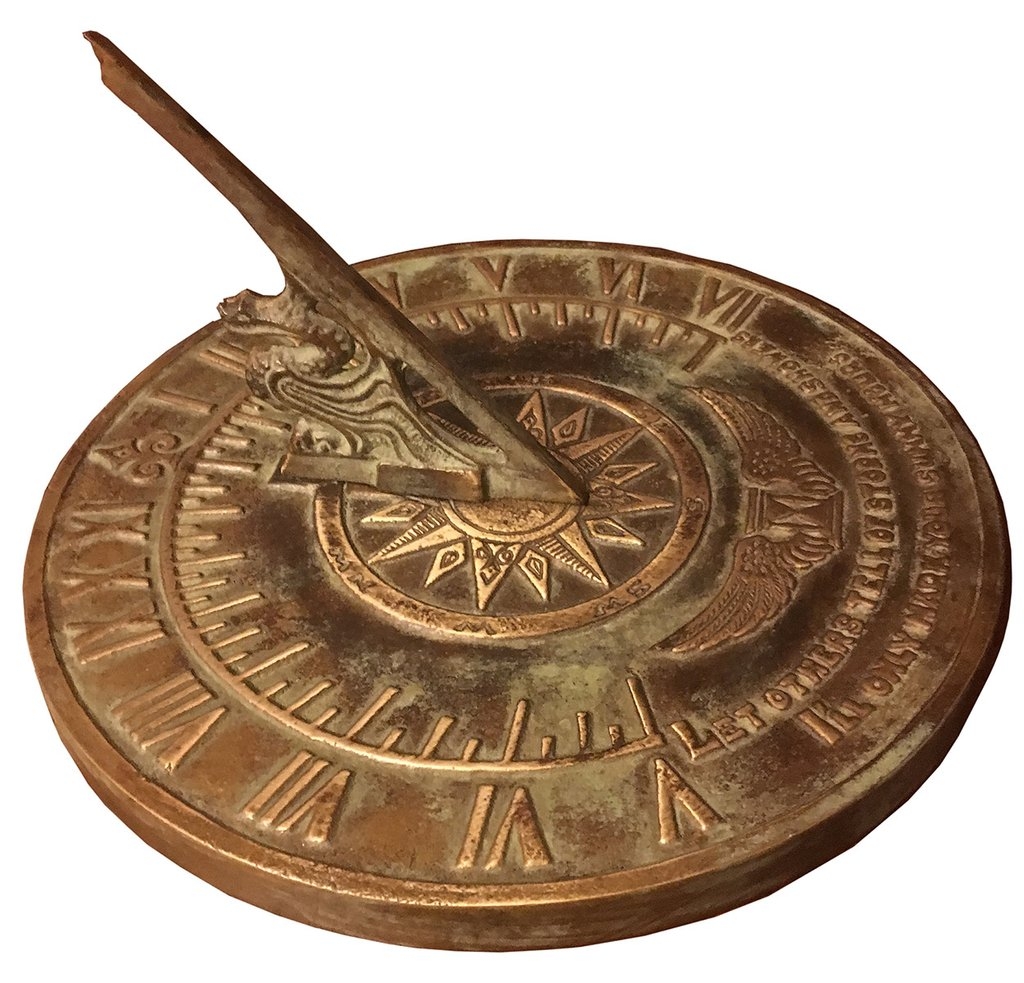In this image, an intricately designed sundial is set against a plain white background, featuring a weathered bronze appearance with golden hues showing through in parts. The sundial is circular, with Roman numerals 1 through 11 engraved around its edge, and a distinctive fleur-de-lis at the position of the 12. At the center of the sundial, an ornate sun is etched, from which protrudes a movable gnomon that points left towards the Roman numeral I. Just below this, on the right-hand side of the dial, is an hourglass with wings, possibly of an eagle, etched with star adornments. This section also bears a partially legible inscription that starts with "let others tell of" and an incompletely visible phrase following "I'll only." The sundial’s intricate details reflect its weathered history, combining the artistry of timekeeping with celestial and terrestrial motifs.